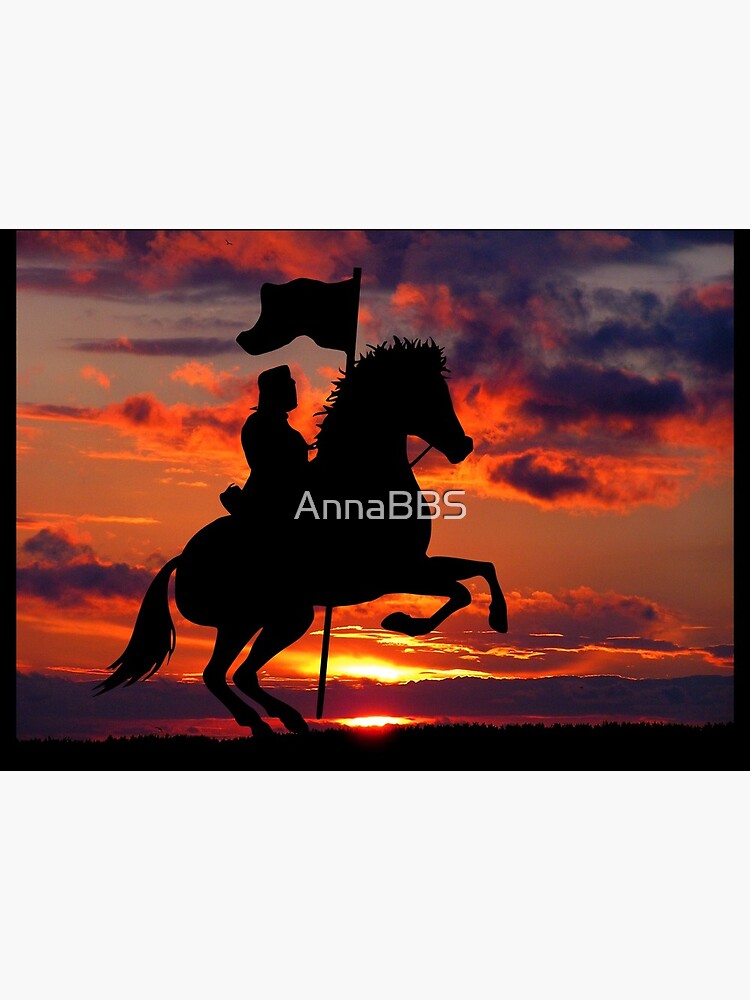The image depicts a striking silhouette of a man on a rearing Mustang horse against the backdrop of a dramatic sunset. The scene captures the powerful moment with the horse's front legs raised, one leg almost touching its belly and the other slightly bent towards the ground, while its tail streams behind. The rider is prominently holding a flag on a long pole, which waves gracefully in the wind. The sky is a captivating blend of pink, orange, and blue hues, with both wispy and puffy clouds tinted by the fading sunlight. The sunset, positioned towards the bottom center of the photo, casts a beautiful glow across the scene, highlighting a possible body of water in the background. The photograph also features text in the center, reading "Anna BBS," which might be a watermark or the photographer's signature.